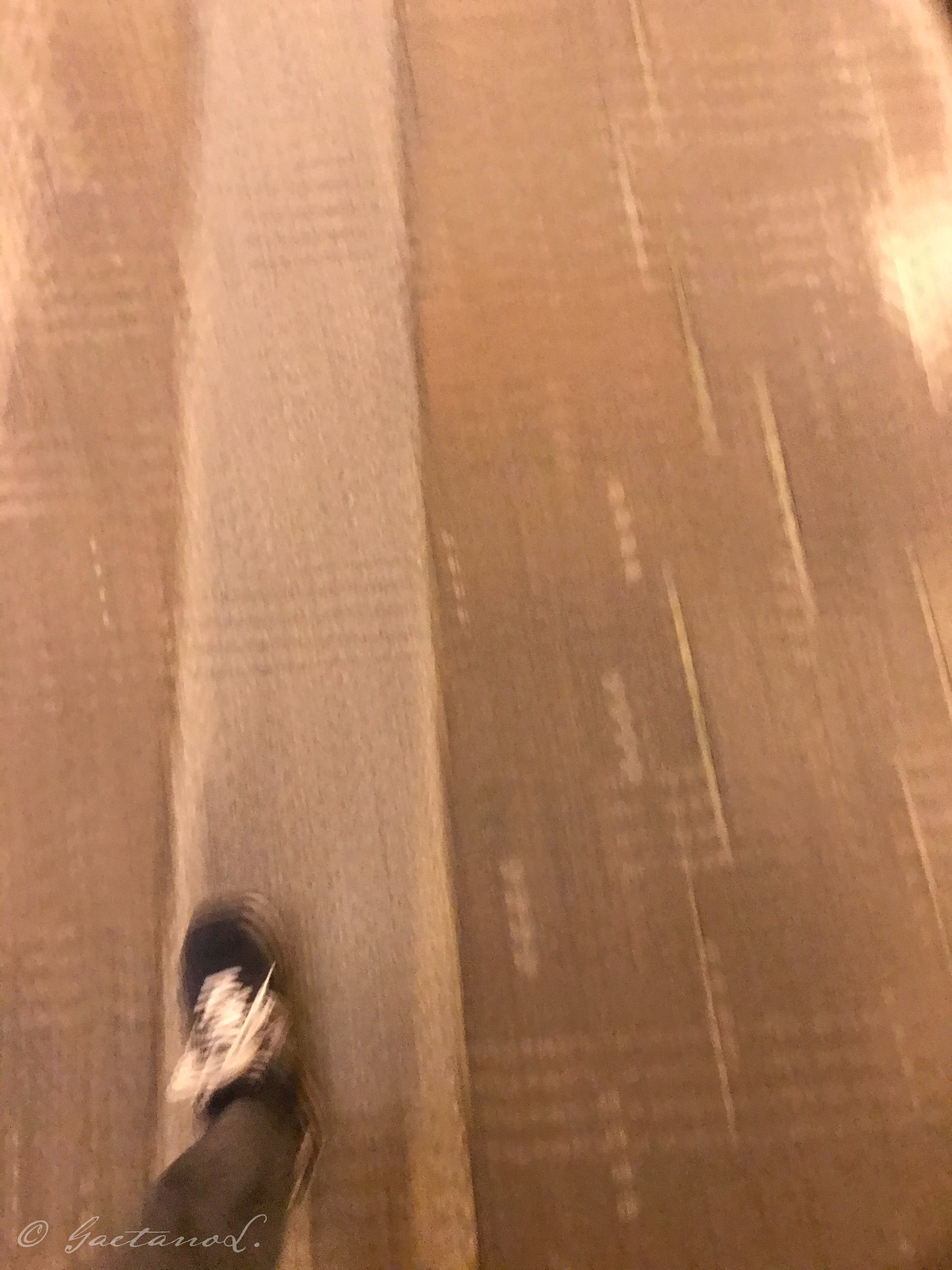The image is a somewhat blurry photograph of a tan-colored floor. In the foreground, at the bottom of the image, a person's left foot and lower extremity are visible. The individual is wearing a blue shoe with a white sole and white shoelaces, paired with gray pants. The shoe appears to be stepping on a vertically oriented lighter brown column on the floor. Adjacent to this column is a section of brown flooring adorned with yellow designs consisting of four dots and horizontally oriented lines. In the bottom left corner of the image, there is a copyright symbol along with the cursive word "GACTANOD."